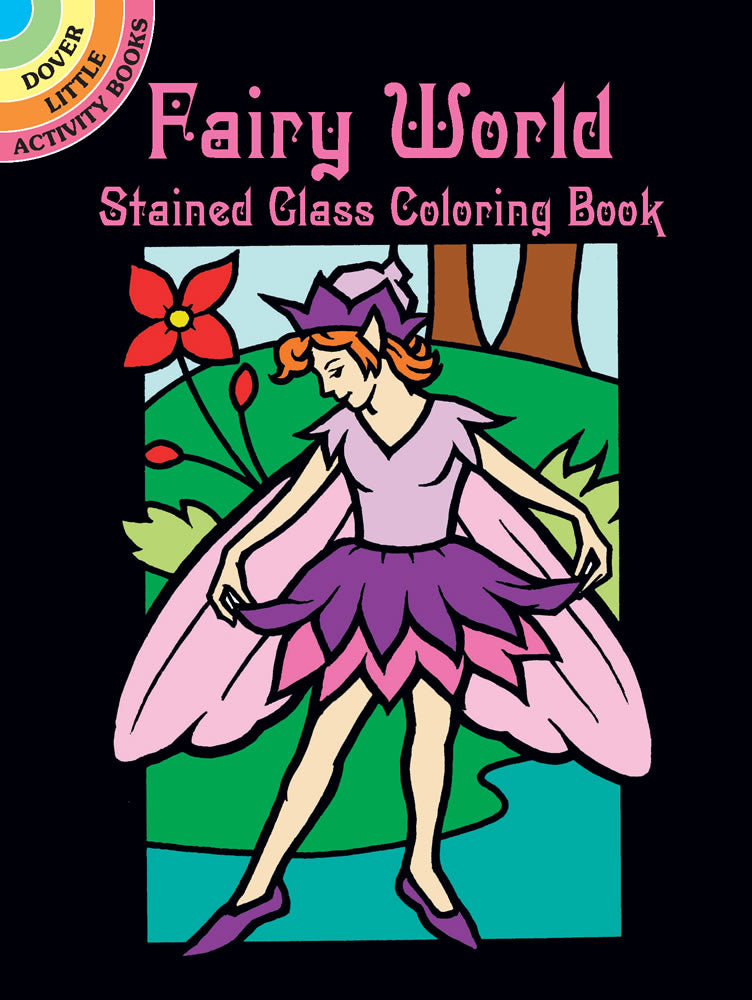This is the cover of a coloring book titled "Berry World Stained Glass Coloring Book," produced by Dover Little Activity Books, identifiable by a quarter-circle rainbow logo in the top left corner. The background of the cover is a solid, opaque black. The central illustration features a female fairy standing near a lake, with a green forest and trees in the background, and a red flower resembling a poppy nearby. The fairy, rendered in a cartoonish style, has bright orange hair and is adorned in a purple hat with a pastel lavender fabric, purples shoes, and a lavender and purple outfit. She has pale skin, pinkish-purple wings, and pointed ears, and is looking down towards her extended right foot. The title "Berry World" is written in bold, decorative pink letters above the fairy, with "Stained Glass Coloring Book" below it.